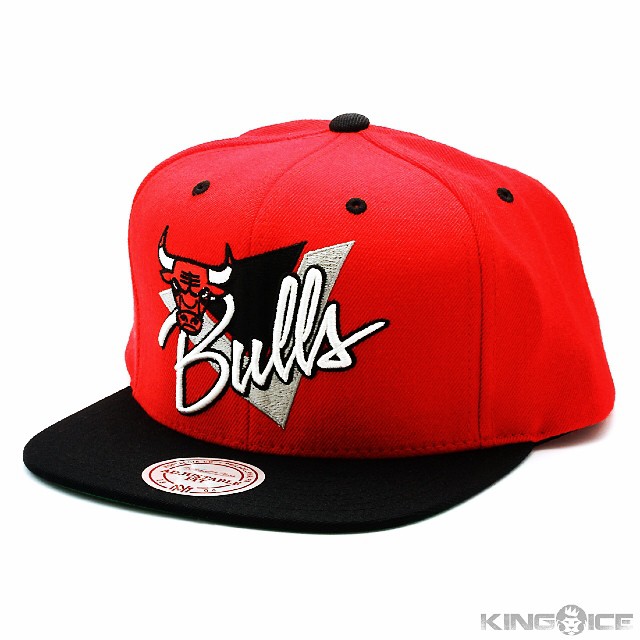Set against a completely white background, this striking Chicago Bulls baseball cap commands attention with its vibrant red body. Featuring a sleek black brim with a prominent white sticker labeled "Adjustable Hat" in red, the cap’s design is meticulously detailed. The top button and ventilation holes are contrastingly black, adding a touch of depth. The face of the cap proudly displays the word "Bulls" in bold white lettering, accompanied by the iconic Chicago Bulls logo: a fierce red bull with white horns. Positioned behind the logo and inscription is a distinctive design— a black triangle superimposed on a larger silver triangle. Additionally, a round patch on the bill hints at the cap's potential collector’s value. Below, the word "King Ice" subtly indicates the manufacturer's name.